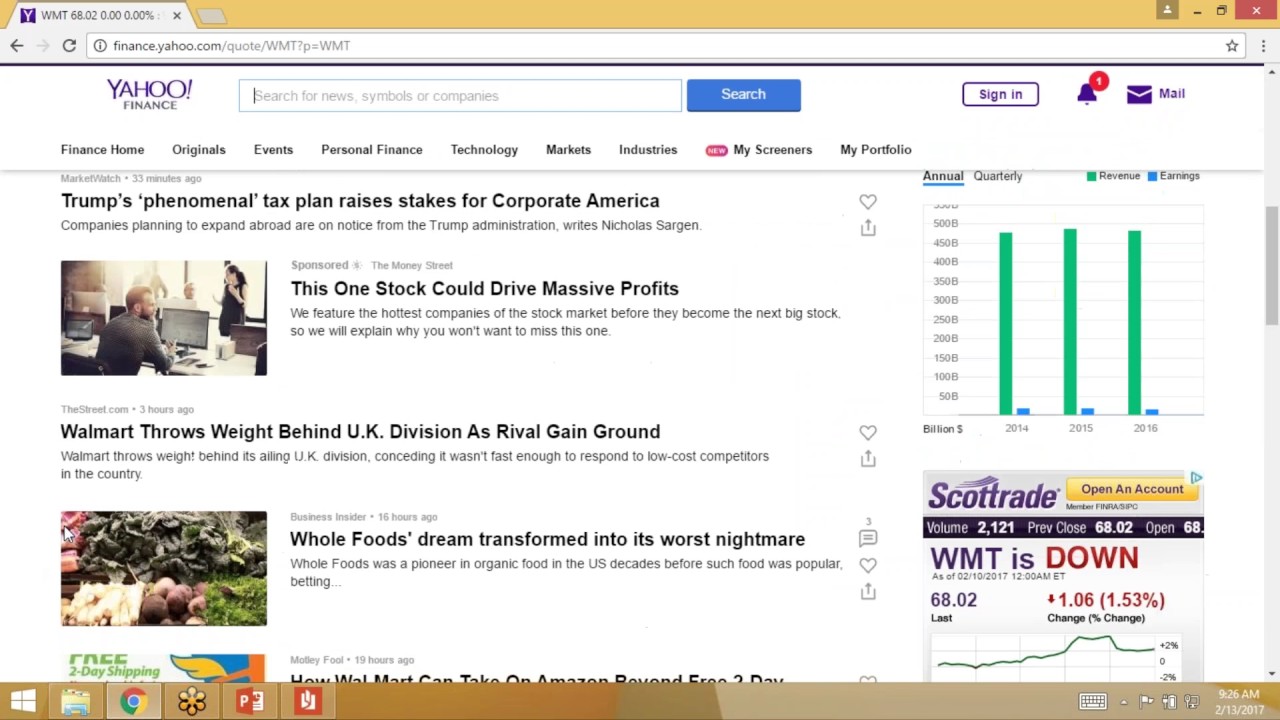The image appears to be a screenshot from the Yahoo Finance website, showcasing various financial articles and features. At the top, the recognizable purple Yahoo logo with an exclamation point is prominently displayed next to the "Finance Home" section. The navigation bar includes options such as Originals, Events, Personal Finance, Technology, Markets, Industries, My Screens, and Profiles, indicating that the user might be signed in and have a personalized experience on the platform.

The main content highlights several financial news articles, including "Trump's Phenomenal Tax Plan Raises Stakes for Corporate America," "Walmart Throws Weight Behind UK Division," and "Whole Foods Dreams Transport and Its Worst Nightmare." These articles suggest the page is densely packed with current financial news and analysis.

There is also a mention of Scott Trade, indicating that the user might be tracking specific stock prices or has integrated financial services into their Yahoo Finance account. Overall, the screenshot captures a multifaceted financial portal, offering a mix of news, personalized finance management, and market monitoring tools.